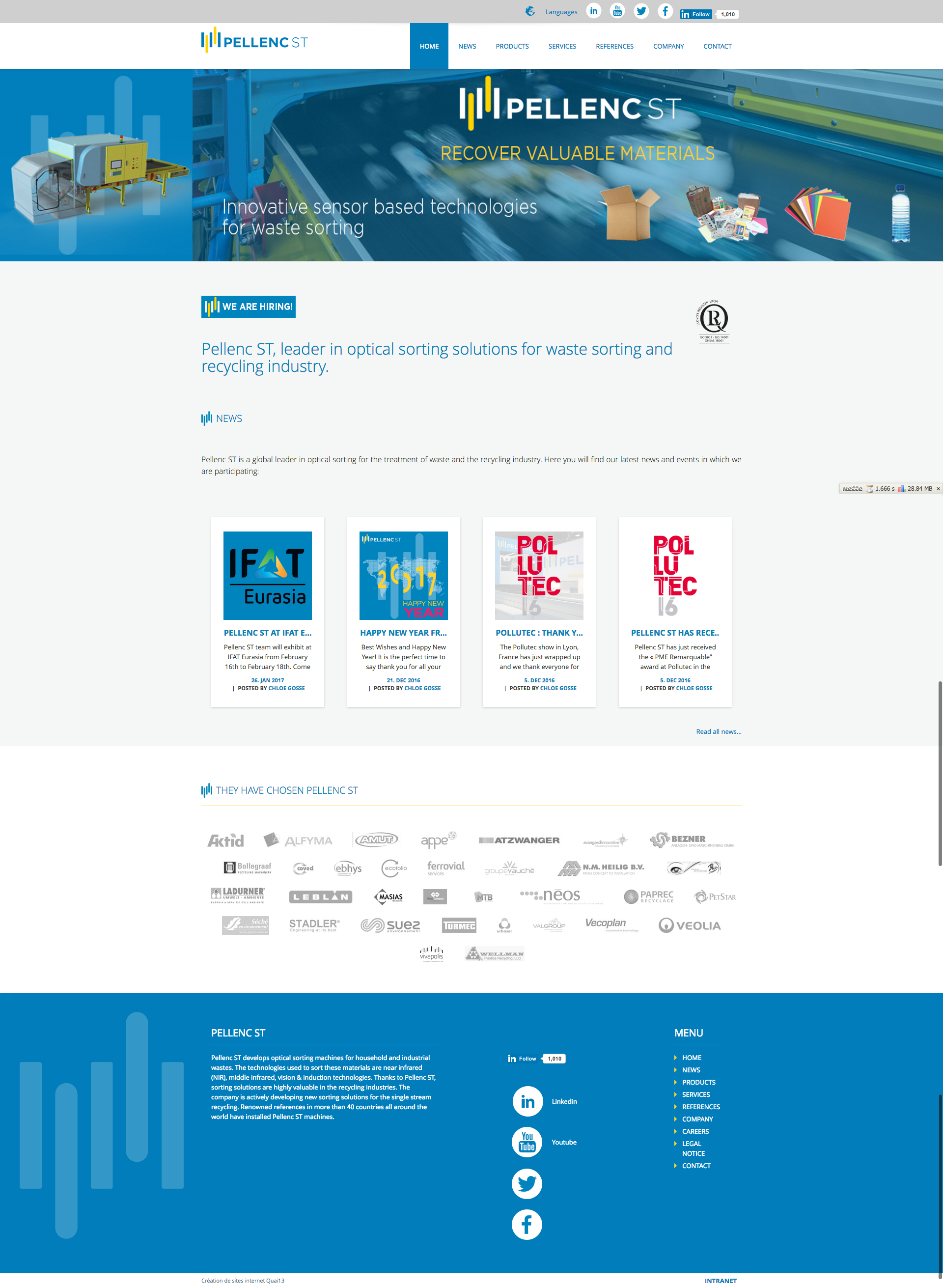The image depicts a promotional webpage for a company named PLINKST. The text highlights PLINKST's focus on recovering valuable materials and innovating sensor-based technologies for waste sorting. The company is currently hiring and is recognized as a leader in optical sorting solutions within the waste sorting and recycling industry. At the top of the page, there are options to change the language and share the content on LinkedIn, YouTube, Twitter, and Facebook, as well as to follow the company's accounts on these platforms. The bottom section displays logos of partners or companies that have utilized PLINKST's services, including AXID, Vekoplan, NIOS, PIPREC, Viulio, and Vesta.